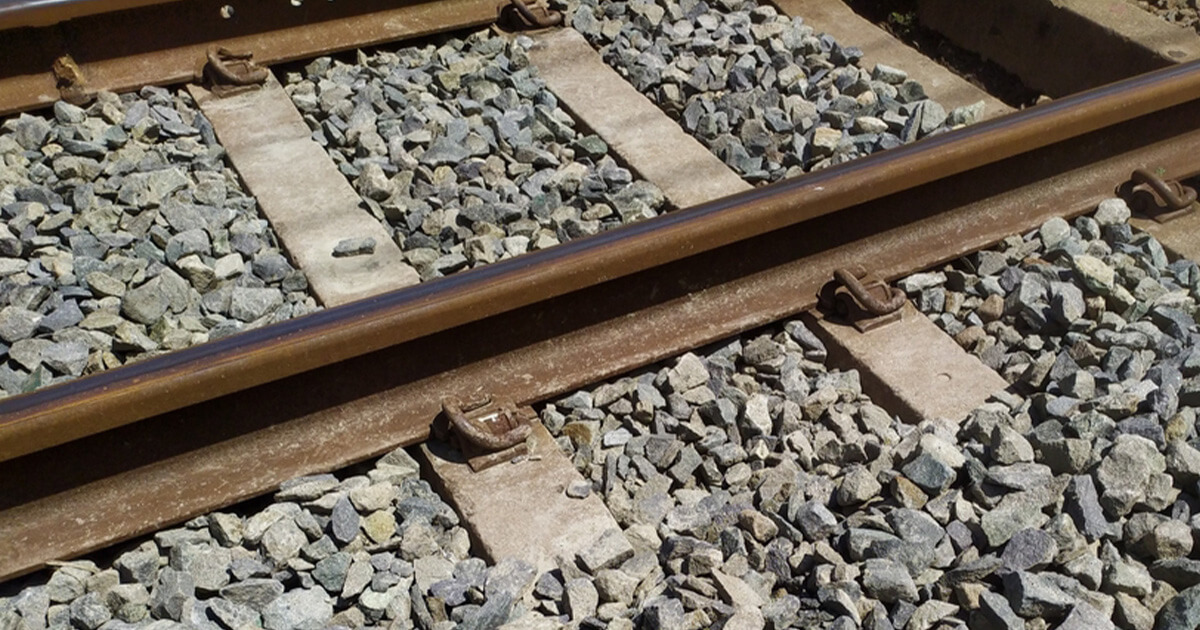The photograph captures a close-up view of train tracks, emphasizing the intricate details of the rails and their support system. The rail in the foreground, positioned centrally, is visibly worn, with bolts and fasteners prominently holding it in place. The track, composed of dark, brown-spotted metal with hints of white, runs diagonally from the bottom left to the top right of the image. Below the tracks, a dense collection of grey and tan rocks of varying shades forms a textured bed. Wooden railroad ties, which are light in color, provide additional support, each firmly anchored by dark brown fasteners. The image, taken in bright, sunny conditions, focuses solely on the tracks and their immediate surroundings, devoid of any background elements such as people or trains. The meticulous close-up and landscape orientation highlight the structural components and the rugged character of the railway.